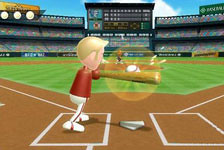The image captures a vibrant moment from Wii Sports Baseball. The scene is set on a stylized baseball field, with a brown textured floor resembling dirt. At the center, a Mii character, sporting white pants and a red shirt tucked into them, stands poised in a batting stance. The character has blonde hair with pronounced sideburns, and is gripping a bat to the right. A baseball is mid-strike, glowing brightly as it connects with the bat, casting dynamic shadows on the home plate.

The field features the traditional layout: a green pitcher's mound at the center, and the expansive stadium with multicolored seating—green, red, and blue—encircling the field. In the top left corner of the image, the game interface displays three balls, denoted by circles filled sequentially. On the top right, a green counter or indicator is visible, and a scoreboard rests at the very top, overseeing the entire scene. The atmosphere is one of excitement, capturing the essence of a pivotal moment in a virtual baseball game.